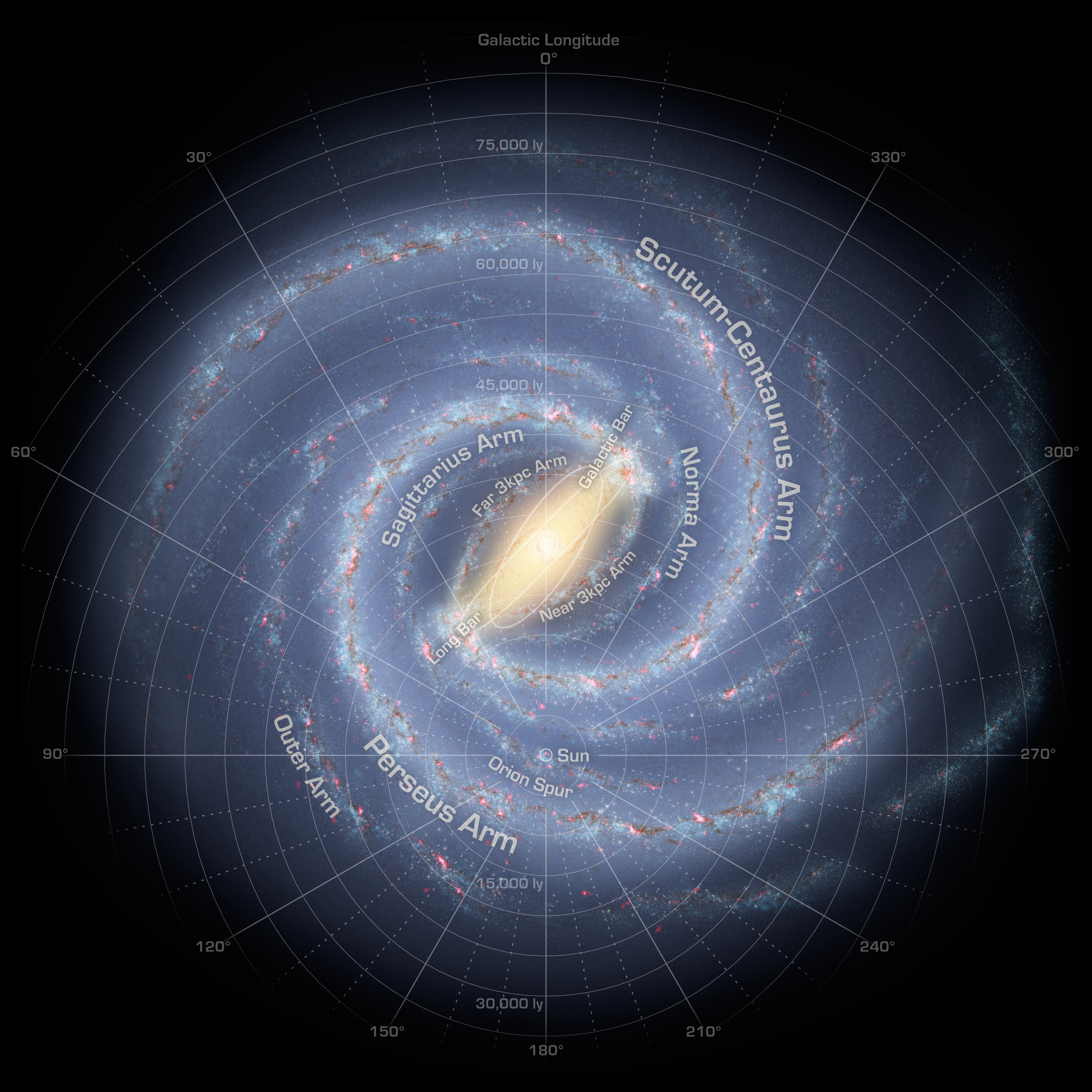The image features a detailed, graph-like illustration set against a pitch-black background. At the center of the image, there's a focal point labeled "The Sun," from which lines radiate outward, similar to the slices of a pie. These radiating lines are marked with degrees, starting from 300°, extending to 330°, 0°, and then continuing in 30-degree increments up to 270°. The diagram is annotated with labels such as "Galactic Longitude," and notable features within the galactic structure are highlighted.

Prominent parts of the galaxy are marked, including "Iron Spur," "Galactic Bar," "Sagittarius Arm," "Scutum-Centaurus Arm" (evoking a mystical, perhaps Hogwarts-like sound due to its complexity), "Perseus Arm," and "Outer Arm." The illustration depicts a majestic, spiral form that resembles the Milky Way, with a nebulous appearance overlaying the graph to visually represent distances and positions within the galaxy.

The image includes specific measurements, showing distances marked as "15,000 LY," "60,000 LY," "45,000 LY," and "Near 3K PC Arm," indicating light-years and parsecs. These annotations provide a sense of scale and spatial relationships within the galaxy, combining scientific precision with the beauty of the Milky Way's structure.